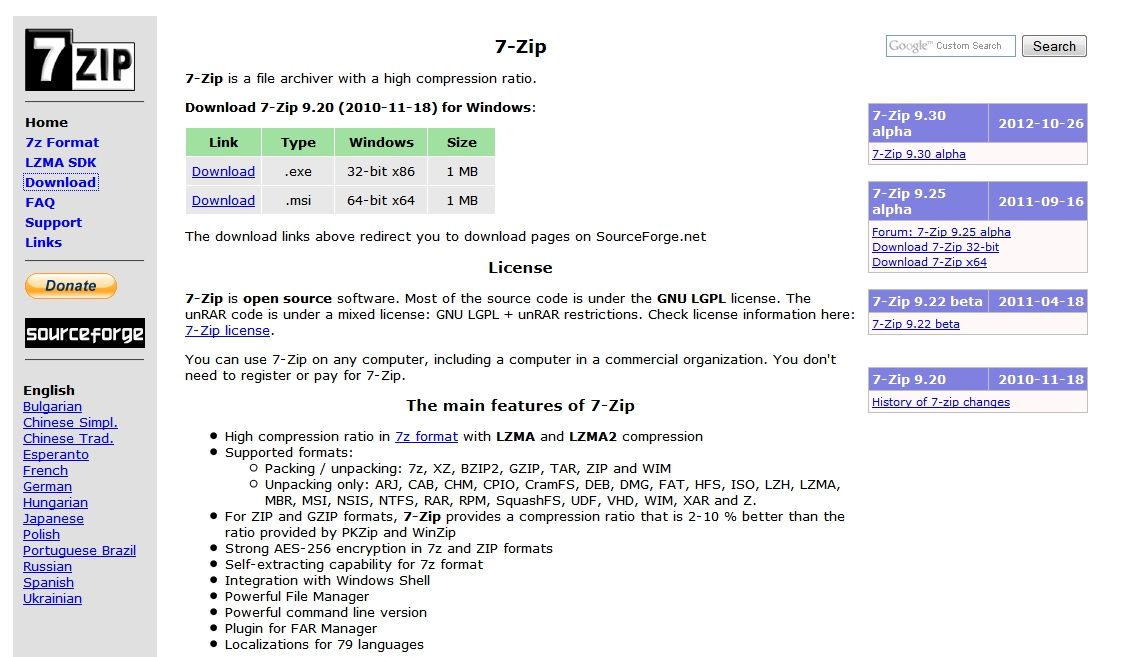This webpage showcases 7-Zip, a versatile file archive software that specializes in unzipping and zipping files, effectively serving as an archive manager. Prominently displayed in the upper left corner is the 7-Zip logo, which features the number "7" against a black background and "zip" written in black on a white background.

The toolbar on the left side of the page includes several navigational links starting with "Home," the current page, followed by "7-Z Format," "LZMASDK," "Download," "FAQ," "Support," and "Links." Beneath these links is a yellow "Donate" button, and directly below it is a link to the SourceForge website. At the bottom of the toolbar, users can choose from various languages to view the website in their preferred language.

Centrally located on the page is a download box offering two distinct links: one for the 32-bit 7-Zip EXE file and another for the 64-bit 7-Zip MSI file. The webpage further provides comprehensive details about 7-Zip, including its open-source licensing information and key features of the software.